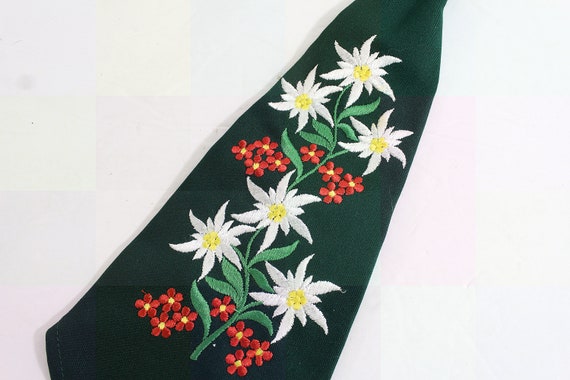This photograph features a dark green decorative napkin positioned against a light gray background, forming a tapered, almost triangular shape that suggests it could also be a tie. The napkin is intricately embroidered with two sets of three symmetrical white flowers, each boasting about ten petals of varying lengths and yellow centers. Interspersed among these are smaller orange flowers, each with five petals and yellow centers. The careful stitching along the edges adds a refined touch to the napkin's overall aesthetic, highlighting its ornate floral pattern.